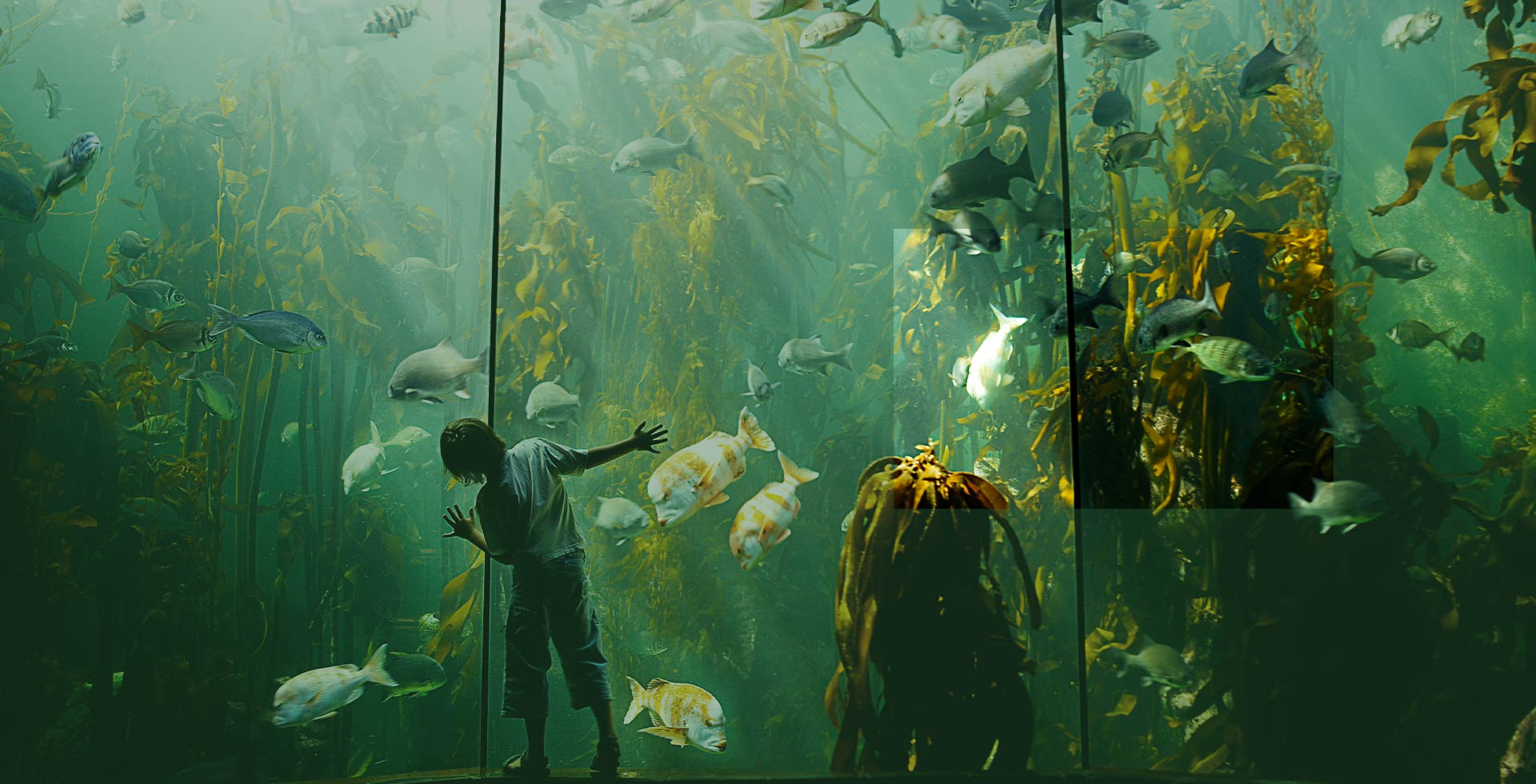In this vibrant color photograph, a young boy stands pressed against the glass of a large aquarium, his small hands placed eagerly on separate glass panes as he gazes at the aquatic life before him. The aquarium exhibits a mesmerizing underwater world, reminiscent of a water jungle, with a green hue permeating the water and rays of light filtering through, mimicking sunlight. Majestic strands of kelp or seaweed stretch towards the surface, creating a lush backdrop.

The scene is divided into three main panels. The first glass pane, where the boy's attention is fixed, features tall water plants and a lively array of fish, including striking orange and white striped ones, as well as black and white, silver, and blue specimens. The middle section, which has a large yellow plant almost as tall as the boy, appears particularly clear and vibrant, showcasing a diverse collection of fish in shades of blue, yellow, and white.

In the far-right panel, another substantial yellow plant dominates the view, though the water here looks slightly more opaque, making the predominantly white and gray fish harder to discern. The overall effect is a captivating snapshot of marine life, evoking curiosity and wonder through the eyes of the young boy engrossed in the aquatic display.